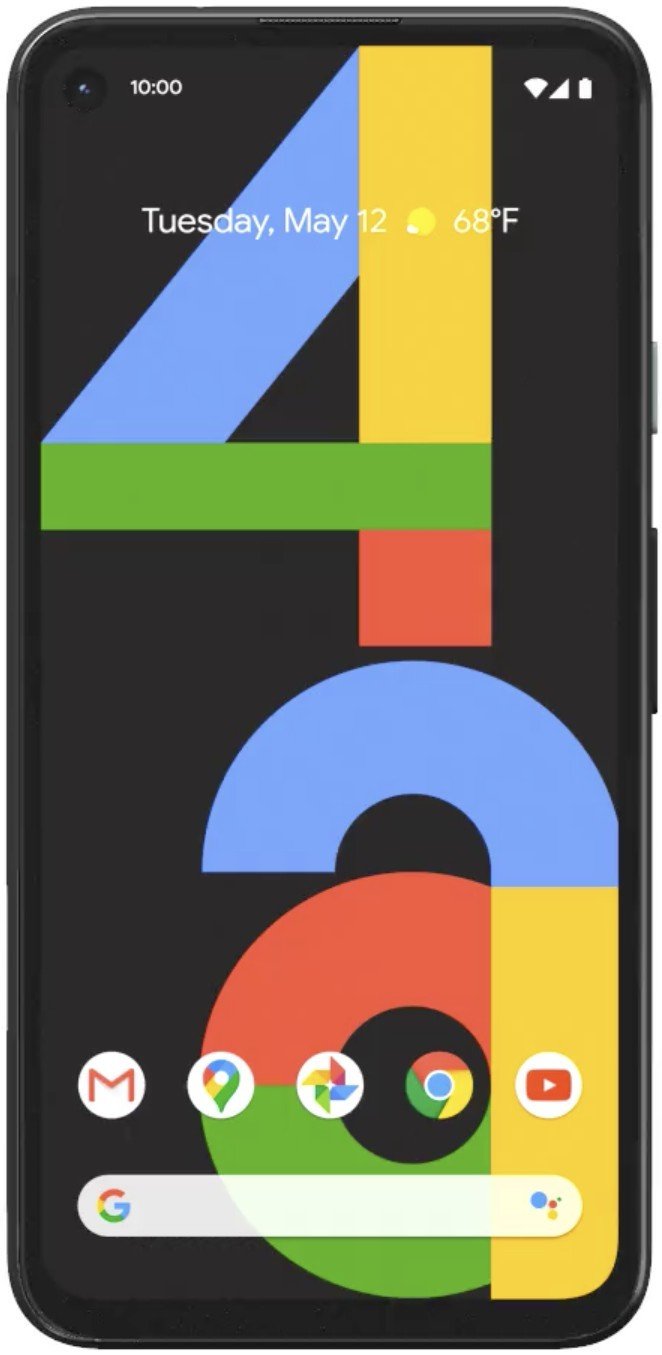The image features a Google Pixel 4A smartphone, characterized by its dark gray, almost black exterior with a reflective, shiny finish that adds a subtle gray tint. The border surrounding the screen is a deeper black, creating a stark contrast with the outer edge. On the right side of the device are three buttons: a large volume rocker and a smaller power button positioned above it.

The phone's display showcases several key details. At the top left corner, an inconspicuous front-facing camera lens sits next to the time, which reads 10:00. The upper right corner displays three fully illuminated icons indicating Wi-Fi connectivity, cellular data, and battery life. The wallpaper prominently features a multicolored "4A," reflecting the phone's model, rendered in Google’s signature blue, green, yellow, and red hues.

The home screen itself displays the date, "Tuesday, May 12th," along with a weather icon showing sunshine and a temperature of 68°F. Towards the bottom of the screen, there are several app icons, including Gmail, Google Maps, Google Photos, Google Chrome, and YouTube, as well as a Google search bar at the very bottom.